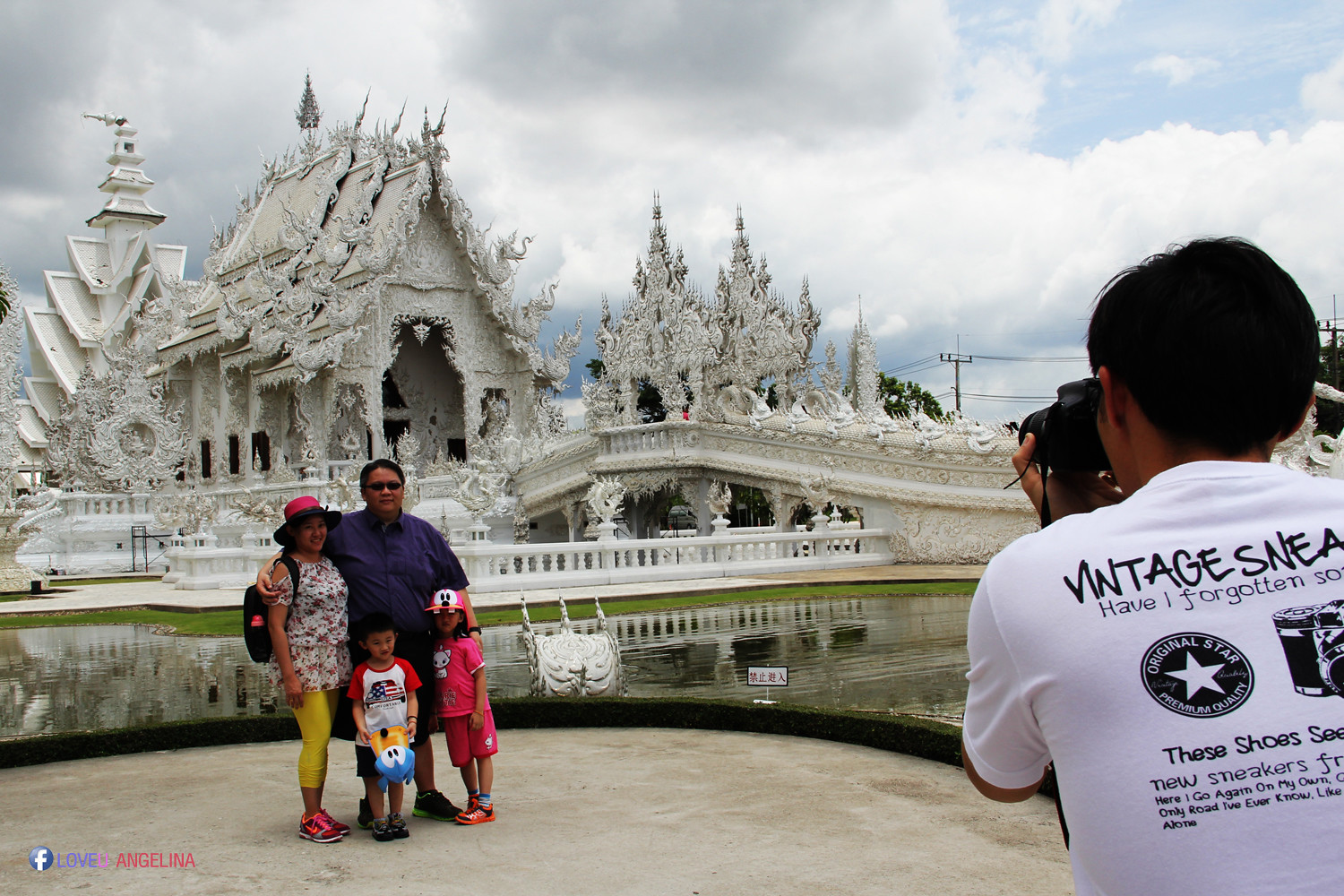A picturesque scene captures a photographer on the right side of the frame, taking a photo of an Asian family standing on the left in front of a majestic white castle. The elegant castle, designed with sharp peaks and intricate details, emanates an off-white hue, almost resembling a frosted gingerbread structure. It stands proudly behind a serene body of water, potentially a pond or a river, over which a graceful white bridge arches. The scene is further adorned by large white clouds in the sky, enhancing the dreamy atmosphere.

The family consists of a man wearing a purple shirt and sunglasses, a woman dressed in yellow leggings and a top, and two young children under the age of five. The little girl is donning a whimsical Goofy hat, while her brother carries another hat in his hand. Their tennis shoes add a touch of casual comfort to their attire, hinting at an adventure-filled day, possibly at an international Disney park. The photographer captures this heartwarming moment as the family stands against the fairytale-like backdrop of the ornate white castle and its tranquil surroundings.